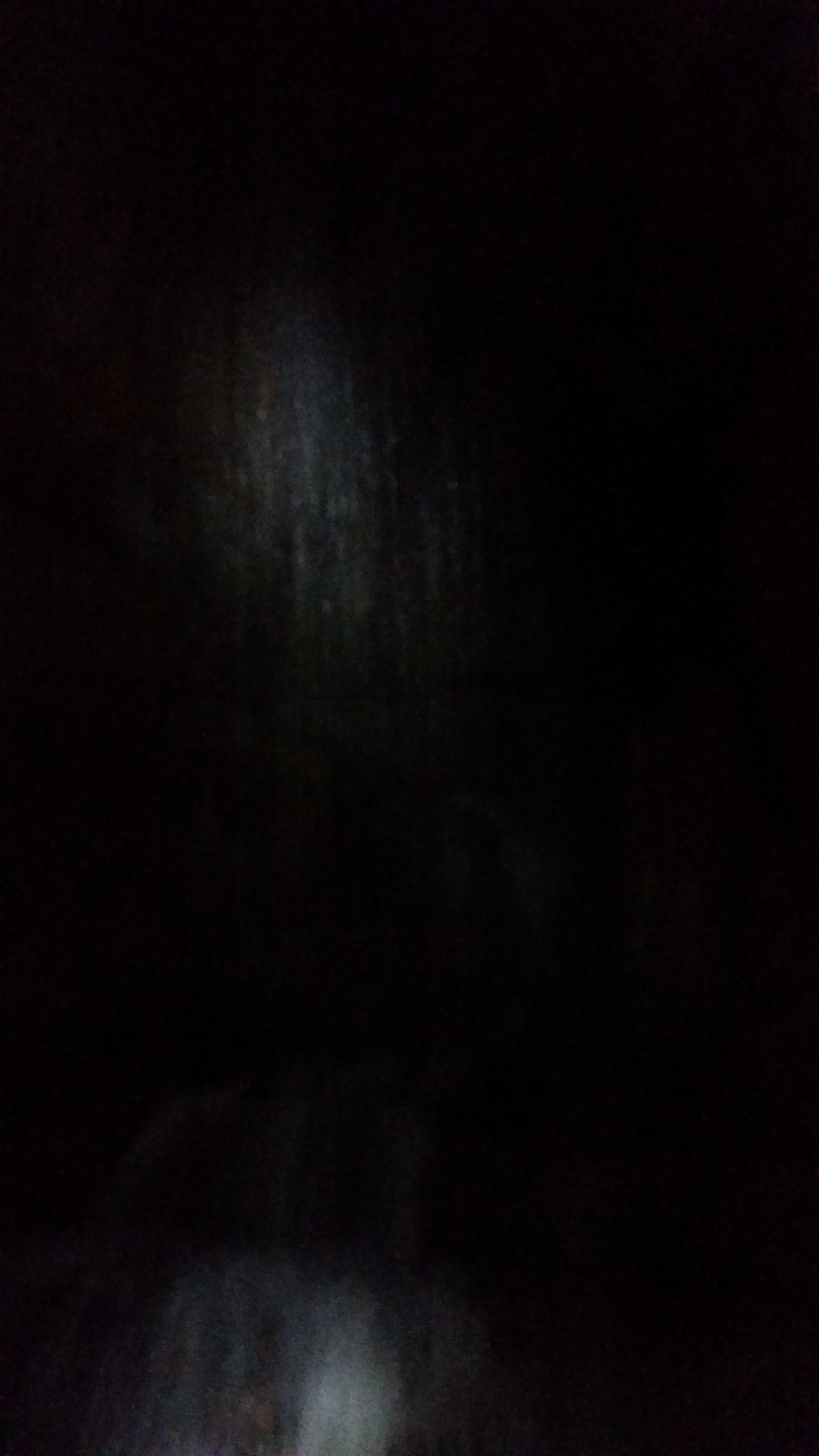This photograph, whether taken indoors or outdoors, is shrouded in darkness, with approximately 90-95% of the image consumed by blackness. The details are sparse, but notable. In the upper left quadrant, just off-center, there is a faint, oval-shaped white object with undefined edges, barely discernible against the dark background. Near the bottom edge, slightly to the left of center, another white object appears, slightly brighter than the first, with softened edges that gradually fade into the black. The photograph is grainy and blurred, without any text or markings. Despite adjusting the contrast to reveal additional details, the image remains overwhelmingly dark, punctuated only by these two subtle white hints.